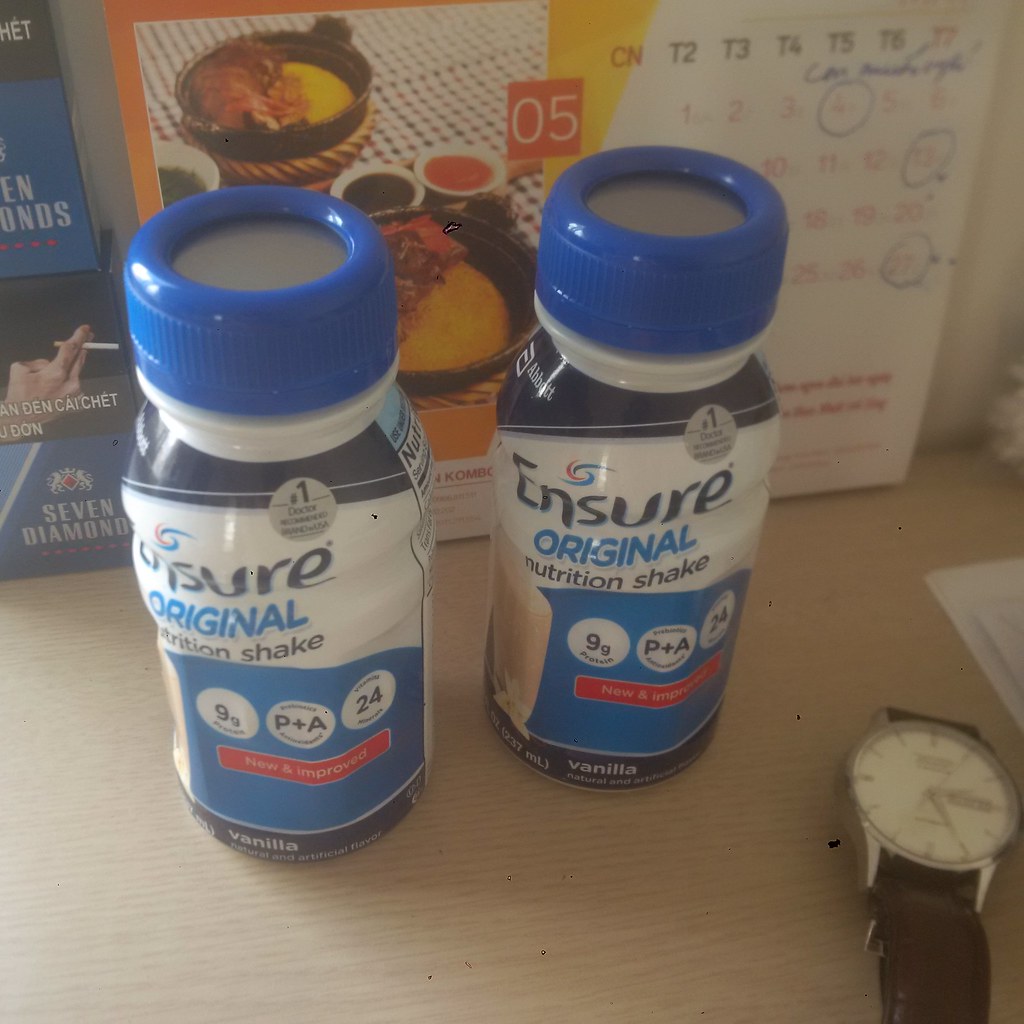The image features two bottles of Ensure nutritional shakes placed on a tan counter. Situated behind the bottles is a calendar displaying images of food, possibly omelets. Specific dates on the calendar, including the 4th, 12th, and 27th, are circled.

The two Ensure bottles, which both contain vanilla-flavored shakes, are central in the image. Each bottle is topped with a blue cap and features a white and blue label. The label details nutrition information in three circular sections at the bottom, set against a blue background. Above these circles, a red bar with the text "New and Improved" can be seen. The word "Vanilla" is highlighted on a darker blue strip at the very bottom of the label. 

On the left side of the photo, there is a watch showing the time as 3:25.